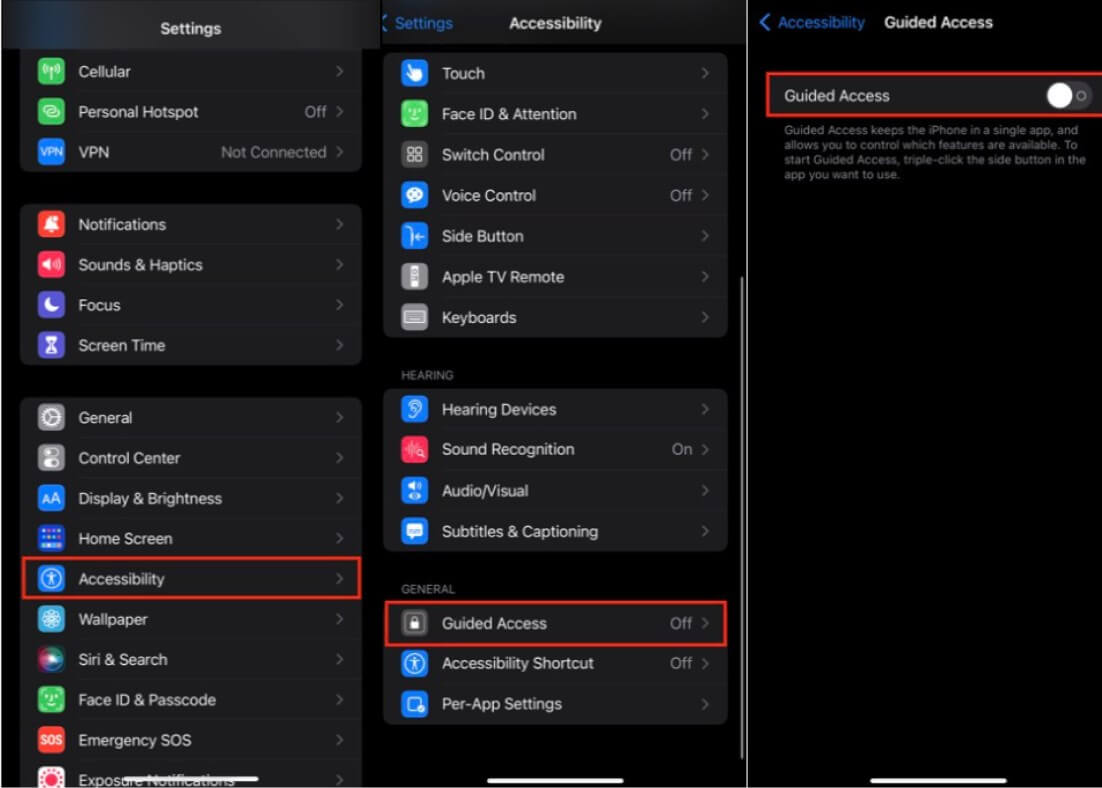This is a color photograph of a webpage with a black background, divided into three distinct sections. At the top of the page, the header is segmented into three parts: on the left, it says "Settings"; in the middle, it says "Accessibility"; and on the right, in white font, it says "Guided Access." Additionally, to the left of "Guided Access," there is the word "Accessibility" in blue font along with a blue arrow pointing to the left.

The content of the page is organized into two long columns and an additional section on the right. The far left column and the middle column extend from top to bottom, containing dark gray rectangles, each labeled with names of various settings and accompanied by colorful icons.

In the far left column, from top to bottom, are items such as "Cellular," "Personal Hotspot," and "VPN." Each of these items has a colorful square icon next to it: both "Cellular" and "Personal Hotspot" have green icons, while "VPN" has a blue icon. The list continues with items such as "Notifications," "Sounds & Haptics," "Focus," and "Screen Time."

The middle column is headed by "Accessibility" and lists items in white font, including "Touch," "Face ID and Attention," "Switch Control," and "Volume Control," among others. Each item in this column also features colorful square icons, in shades of blue, green, and gray.

On the right side of the page, under the headline "Guided Access," the section is highlighted by a red rectangle outline. Beneath this heading, there is a description in white font that reads, "Guided Access keeps the iPhone in a single app," with further information continuing below this introductory phrase.